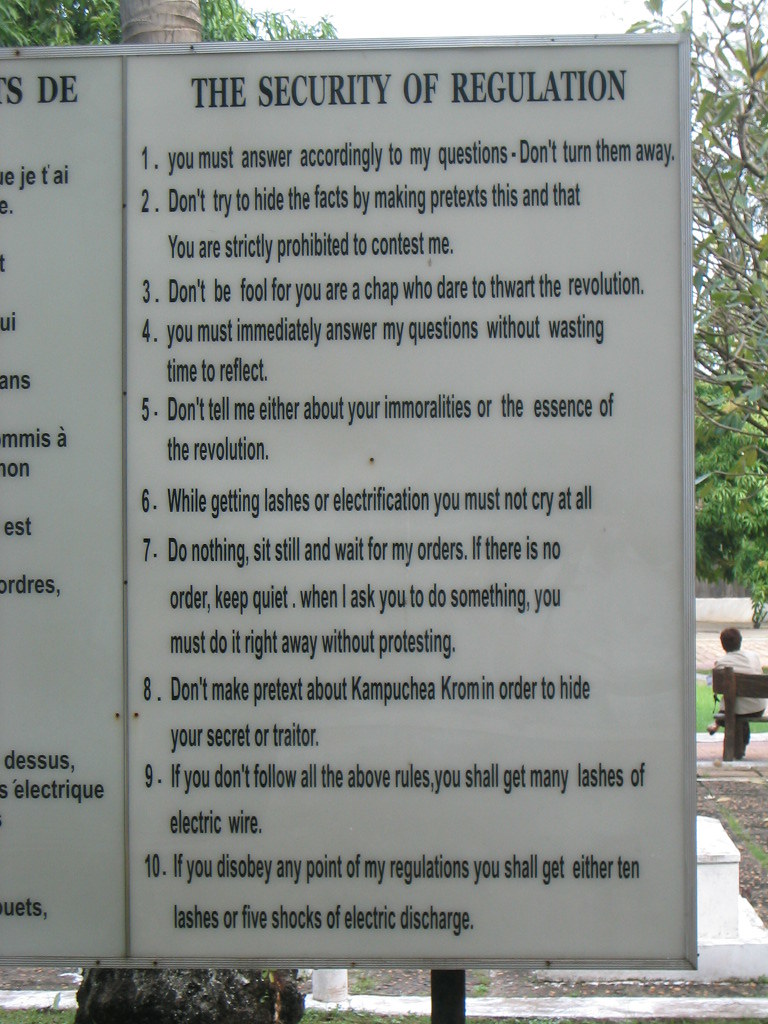The image captures a detailed view of a plaque outlining Khmer Rouge security regulations. Positioned outdoors, the plaque features an off-white background with black and white text. Its title reads "The Security of Regulation," followed by a list of these stringent rules. The first rule states, "You must answer accordingly to my questions. Don't turn them away," while the last rule warns, "If you disobey any point of my regulations, you shall get either 10 lashes or five shots of electric discharge." The plaque contains a total of 10 points, emphasizing the draconian measures enforced during the Khmer Rouge regime. The setting appears to be a park, as evidenced by surrounding benches, trees, and glimpses of white stairs peeking from behind the plaque. In the background, one can faintly discern the back of a person seated on a bench, adding to the somber atmosphere of the scene.